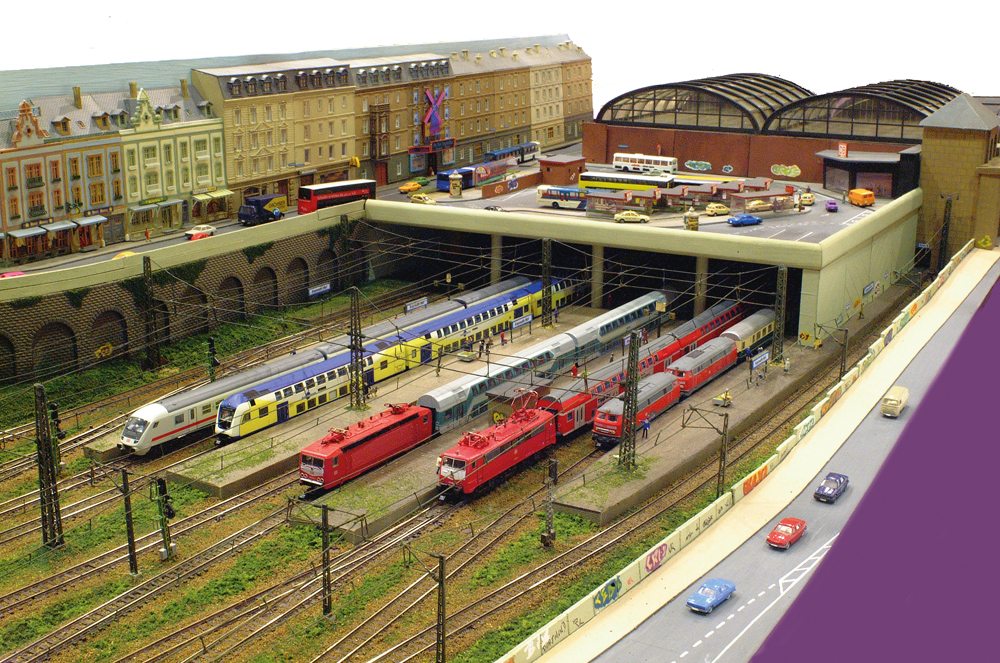This detailed image depicts a highly realistic model of a train station, intricately crafted to showcase the bustling environment of a transportation hub. In the foreground, there is an expanse of about 8 to 10 parallel train tracks laid out on a grassy terrain. Interestingly, the area directly beneath the tracks is a contrasting brown, perhaps simulating worn, heavily-used ground. 

Positioned along the tracks are five meticulously detailed model trains. Each track is bisected by concrete platforms, providing realistic spaces where passengers would board the trains. On the rightmost track, a vivid red train consisting of three cars stands ready. Adjacent to it, another red train is slightly longer, extending to about four cars. Following these, there is a train that features a red lead car with subsequent cars painted in white and blue. Next in line is a train adorned in yellow and blue hues, while the final train presents a sleek, modern appearance in white and gray tones.

All the trains appear to be emerging from a dark, tunnel-like structure supported by robust pillars, suggesting the trains are passing underneath a raised area. This upper level seems to serve as a parking lot, an entryway, or even a roadway, as evidenced by the presence of a stationary bus.

To the left of this intricate train scene is a replica of an urban setting with detailed model buildings that breathe life into the miniature layout. On the right side of the station, a single-lane road features four small model cars, enhancing the realism. Adding to the urban feel, there is graffiti art carefully applied to the model walls adjacent to the sidewalk. 

Furthermore, the scene is dotted with electric poles, strung with numerous wires stretching along the tracks, reflecting a detailed commitment to authenticity. The tracks are set in a depression between elevated roads flanking the scene to the left and right. On the left road, in front of the buildings, is an elevated street level, accentuating the depth and dimension of the model.

Notably, a detailed double-decker bus and several brown buildings with distinctive glass roofs add to the immersive environment of this miniature urban landscape.